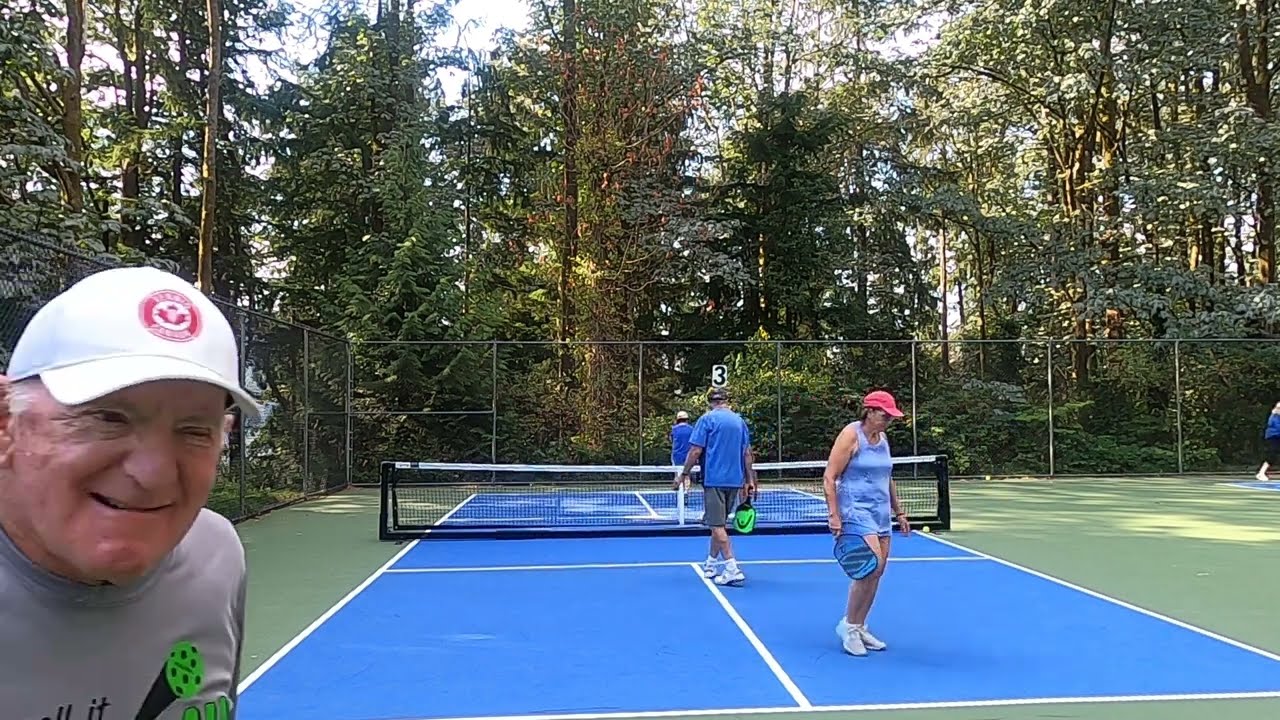The image showcases a vibrant pickleball court bathed in sunlight but shaded overhead by lush, leafy green trees. The royal blue court is accented by green outer sections and enclosed by a sturdy fence. The setting is calm yet lively with people either playing or preparing to play pickleball, evidenced by their paddles. To the immediate left, an elderly man in a grey shirt adorned with a pickleball print and a white hat featuring the Canadian flag grins joyfully at the camera. The playful atmosphere is palpable. In the middle of the court stands a woman dressed in a blue tank top, blue shorts, white shoes, and a pink hat with sunglasses, holding a blue paddle. Adjacent to her, a man in a blue t-shirt, gray shorts, and white tennis shoes grips a green paddle, facing the net. Further in the background, near the far side of the court, another individual, partially obscured, wears a white hat and a blue shirt. A figure sporting a blue shirt and black shorts is just visible on the very right edge of the image, stepping out of the frame. The trees surrounding the court cast gentle shadows, providing a serene backdrop to the lively scene.